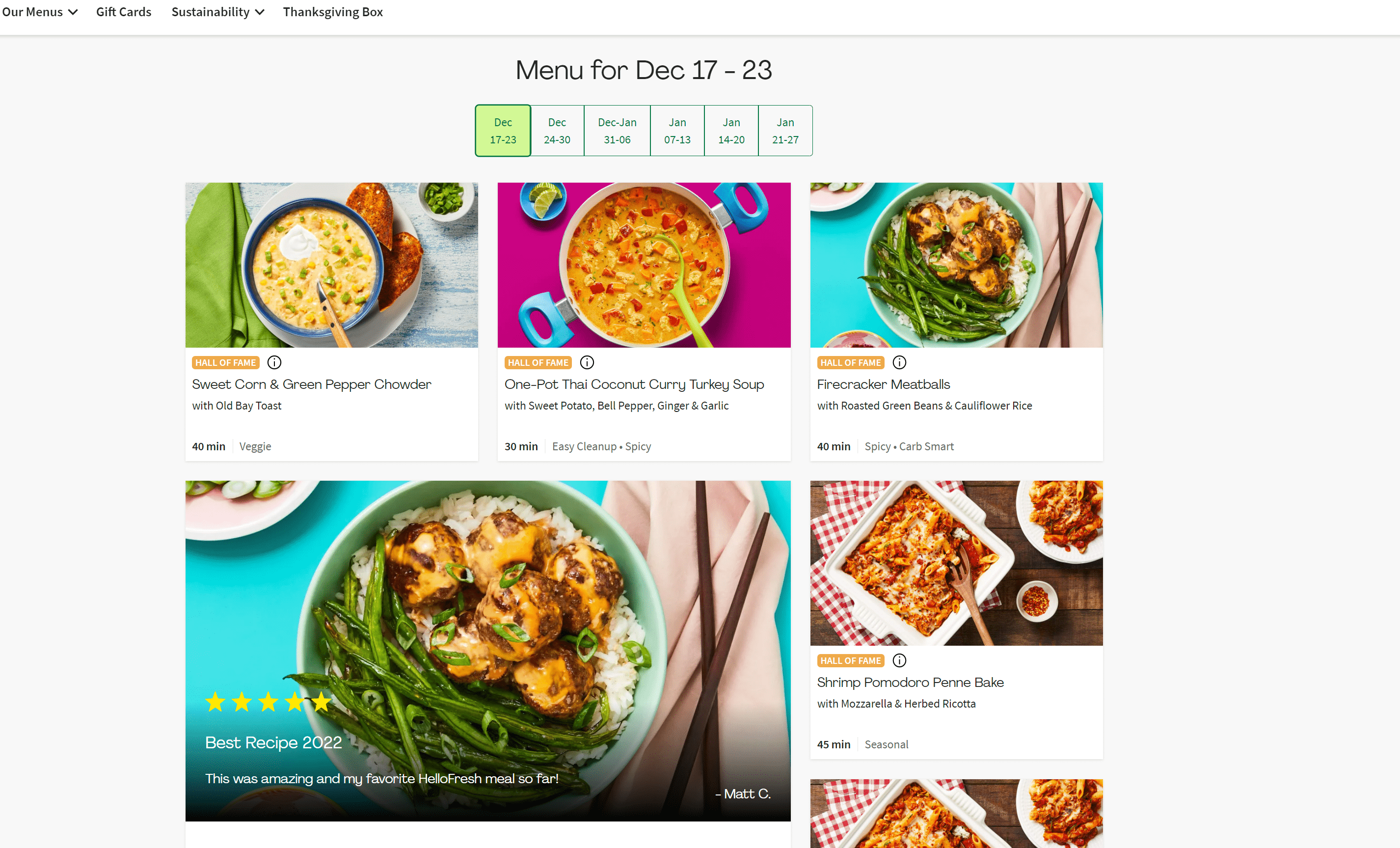The image features a light gray colored background with a detailed layout of a menu. In the upper left corner, the text "Our Menu" is prominently displayed. Below this heading, there is a drop-down menu with options including "Gift Card" and "Sustainability," each accompanied by its respective drop-down box. Additionally, another drop-down box labeled "Thanksgiving Box" is present.

Below these options, the menu for specific dates is outlined. A green box highlights the dates ranging from December 17 to 23. Beneath this, the dates are further extended to December 24-30, December 31 - January 6, January 7-13, January 14-20, and January 21-27. 

Under this date section, images of various dishes are showcased. The top left dish is labeled "Sweet Corn and Green Pepper Chowder with Old Bay Toast." The middle dish is described as "One Pot Thai Coconut Curry Turkey Soup with Sweet Potato, Bell Pepper, Ginger, and Garlic." Lastly, the dish on the right is identified as "Firecracker Meatballs with Roasted Green Beans and Cauliflower Rice."